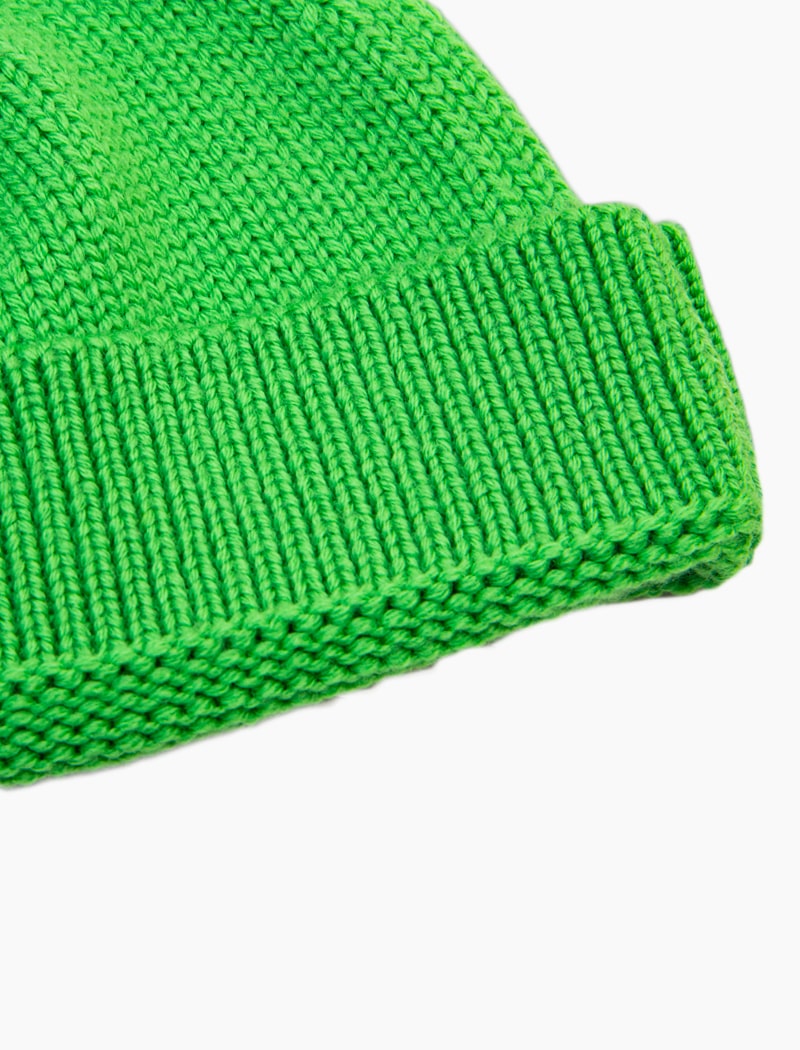This close-up image showcases a beautifully knitted item, likely the bottom corner of a winter wear piece such as a sleeve of a sweater or the edge of a ski hat. The knitting features an intricate arrow pattern where one row of arrows points upwards and the next row points downwards. The yarn used is a light, yellowish-green color, distinct from a dark olive green. The item is placed on an off-white surface and appears to be creased in the middle, suggesting it might be the fold of a cap or a sleeve. The detailed weaving emphasizes the meticulous craftsmanship of the piece, though the image does not capture the entire item, just about 90% of it.